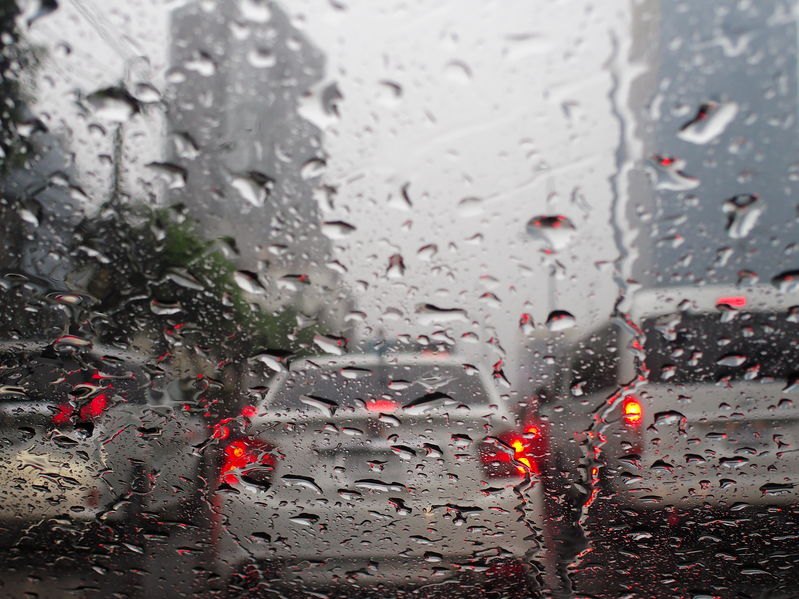The photograph captures a rainy day view through a windshield, adorned with large raindrops and streaks of water running down the glass. Beyond the droplets, the image showcases halted traffic with three rows of vehicles, all displaying red brake lights. Directly ahead, a small compact car with bright red taillights is prominently centered. To the right sits a larger, white minivan, and to the far left, a silver SUV is partially visible. The weather appears foggy, further blurring the details of the scene. In the background, out-of-focus buildings rise on either side, hinting at a city street setting. To the left, a few streetlights and power lines are discernible, alongside a line of trees. The misty atmosphere and wet surface emphasize the damp, overcast conditions of the day.